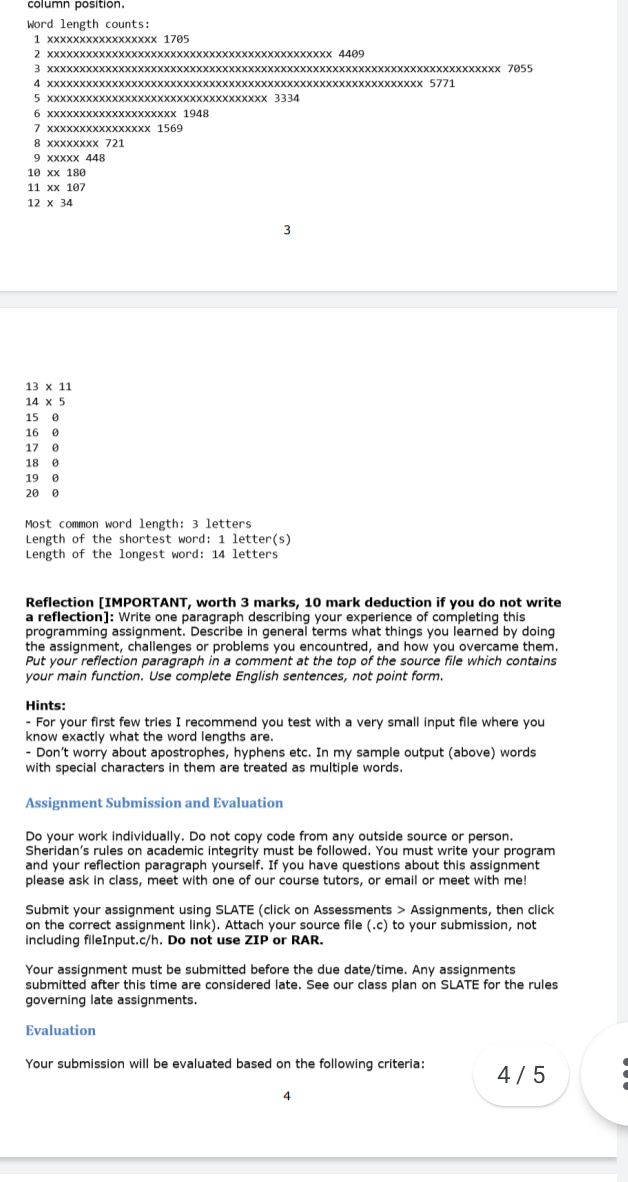**Webpage Screenshot of an Assignment PDF**

The image captures a webpage displaying a PDF file with a white background. The visible section is scrollable through multiple pages, and part of the first page is in view. At the bottom center of this page, the number "3" is prominent. The document appears to detail an assignment, including extensive numerical data and guidelines.

The visible text includes instructions on interpreting "word length counts," represented in a column format. The document lists sequences such as "1 7 0 5 2", followed by various patterns of 'x' characters and numerical values like "4 4 8 0 9 3" and "7 0 5 5." These sequences continue with numbers interspersed between sequences of 'x's: "4 5 7 7 1," "5 3 3 3 4 6," "1 9 4 8 7," "1 5 6 9 8," "7 2 1 9," and so on.

Further, the document outlines informational segments such as "most common words" and specifies data points like "three letters" for "length of the shortest word" and "four letters" for "length of the longest word." Following this, there is a directive for a "reflection" paragraph, instructing the student to write about their experience completing the assignment. This includes discussing the learned concepts, encountered challenges, and solutions implemented. 

Hints for the assignment suggest testing with small input files and mention that special characters in words should be treated as multiple words. 

Submission instructions are formatted with steps: students are directed to submit their assignments via Slate by clicking on "assessments," then "assignments," attaching the source file without using ZIP or RAW formats, and noting the importance of timely submissions.

The document additionally emphasizes academic integrity, reminding students to work individually and avoid external code sources, adhering to Sheridan’s academic integrity rules.

The bottom right of the page displays a faint "4-4-5," likely indicating a reference or pagination detail. The assignment addresses further guidelines under "Assignment Submission and Evaluation," marked in blue text, elaborating on details and evaluation criteria for the submission.